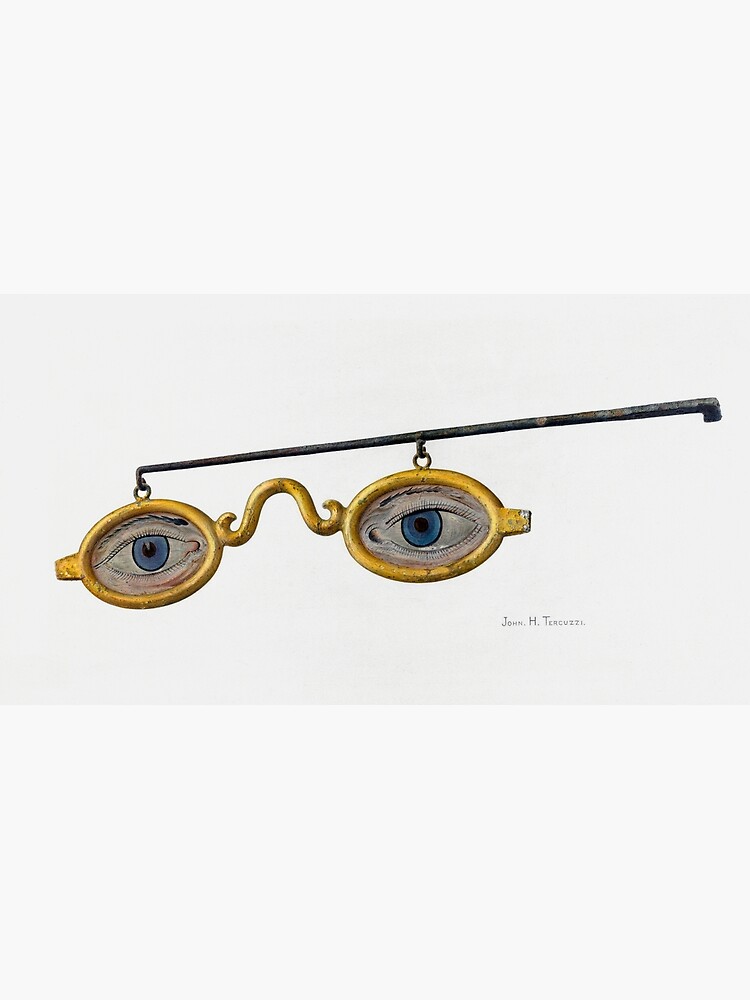This detailed illustration by John H. Tercuzzi, superimposed on a clear white background, features an abstract depiction of a pair of yellow framed glasses. Each lens houses a painted blue eye, complete with detailed elements such as thin black eyebrows and visible eyelashes, adding a semi-realistic touch. The glasses are suspended by a metal pipe or black bar extending horizontally, with a handle-like structure connecting downward. There is a notable arch detail at the nose bridge, indicating an old-world design. The overall frame appears slightly worn with a thick structure. The illustration includes the artist's signature, "John H. Tercuzzi," in the lower right-hand corner, marking it as a completed art piece. Without additional objects against which to scale the size, the white background leaves the dimensions of the illustration ambiguous.